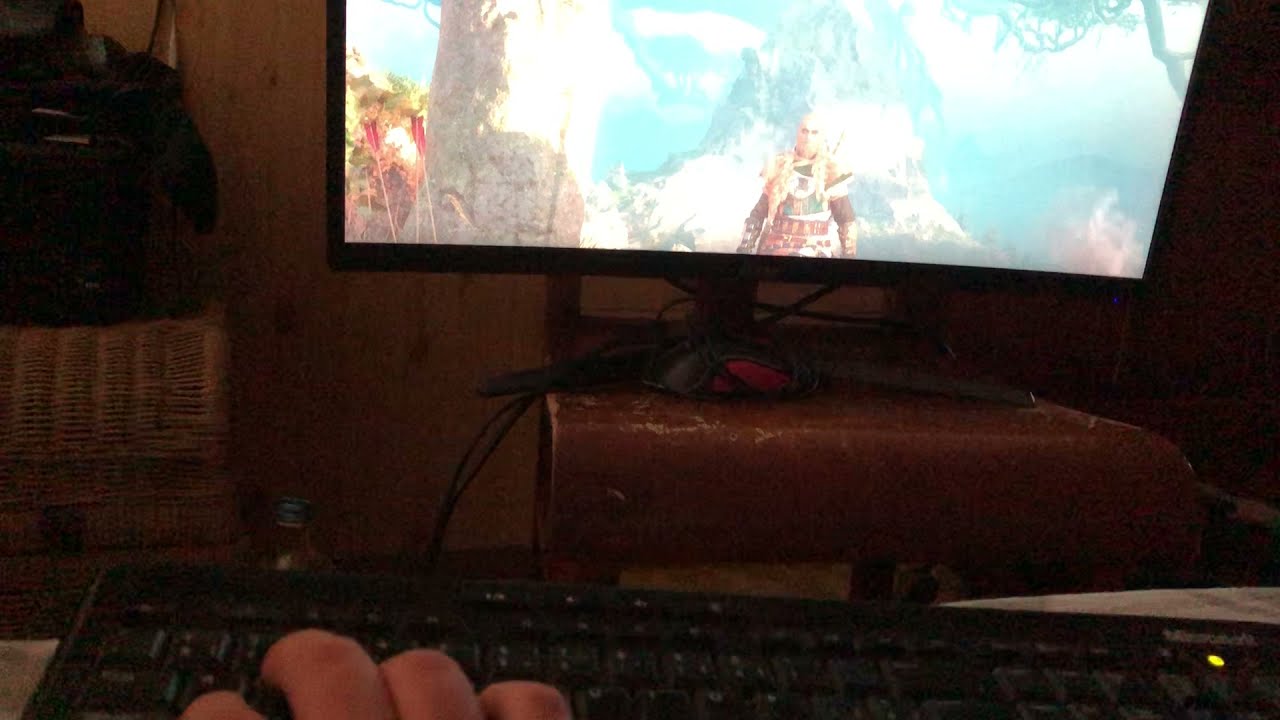The photo depicts a close-up view from the perspective of someone typing on a black computer keyboard, with visible dark-skinned knuckles on the right hand. The computer monitor, positioned atop a worn or old book, displays the lower half of a video game screen featuring a blond-haired elf or warrior with a sword on his back, standing against a mountainous backdrop. To the left of the monitor, there's an identifiable wicker basket, possibly containing some dark objects. The image is somewhat dark, making it challenging to distinguish all details clearly. Underneath the screen, there appears to be some brown material, possibly leather. The keyboard includes a small green light on the right side, marked with "Microsoft." Scattered across the desk are other indistinct items that contribute to the busy scene.